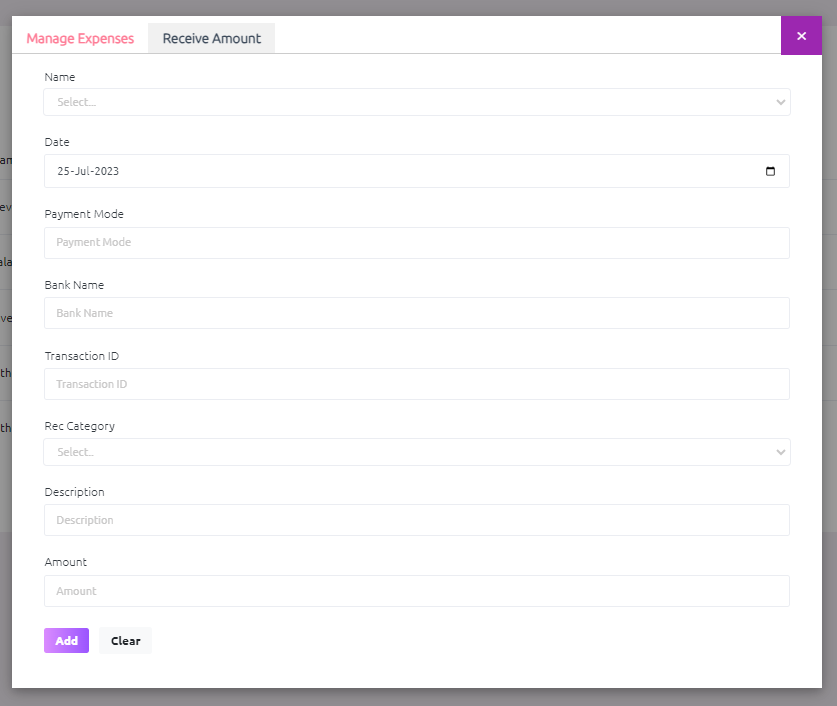The image depicts a pop-up window overlaid on a webpage or application, which is blurred and indistinct behind it. The pop-up window is bordered by a sleek gray frame, creating a clear, defined boundary around its content. Inside the window, which features a clean white background, a prominent purple box with a white 'X' in the upper right corner serves as the close button.

At the top left corner of the pop-up window, the title "Manage Expenses" appears in striking red text, immediately drawing attention. Just beneath this, the phrase "Receive Amount" is displayed in standard black text.

The main body of the pop-up window is dedicated to an expense management form, featuring several labeled fields for user input. These include:
1. "Name" with a selectable drop-down menu.
2. "Date" pre-filled with "25 July 2023."
3. "Payment Mode" 
4. "Bank Name" 
5. "Transaction ID" 
6. "REC Category" with a drop-down menu.
7. "Description"
8. "Amount"

Each field is accompanied by corresponding text boxes for user entries. Below these fields, on the bottom left-hand side, are two command buttons. The first button, colored purple with white text, says "Add." Next to it is a gray button that reads "Clear" in black text, likely intended to reset the form.

Overall, the window presents an organized and user-friendly interface for managing expenses, designed with clarity and accessibility in mind.